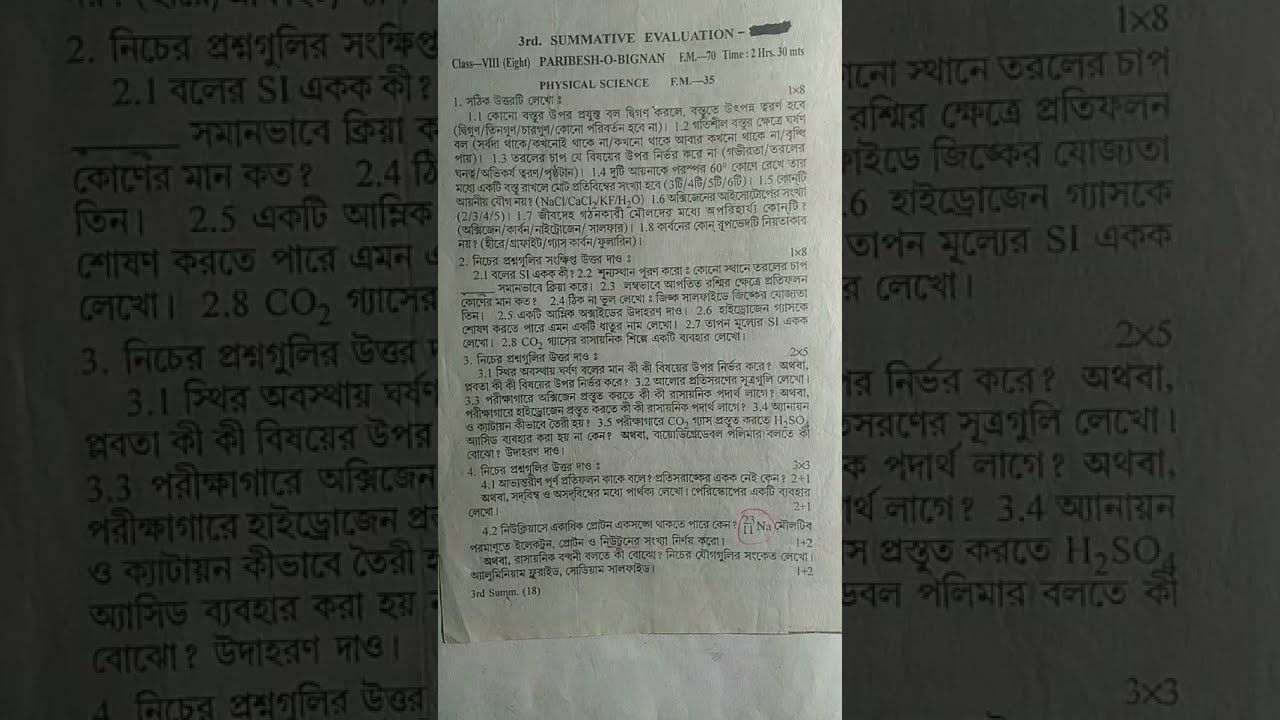The image showcases an off-white paper resembling a receipt, prominently centered against a dark background filled with possibly Arabic or another foreign language text. The title on the paper reads "3rd RD Doc Summative Evaluation" and "Class VIII" is followed by "Paribished-old-biglet" which might be a misinterpretation. Below this, it lists "FM 70, Time 2 Hours 30 Minutes, Physical Science." The paper includes various sections and formulas, with notable ones such as "CO2" and "23/11 NA" circled in red. Toward the bottom, the text includes "GED Summa 18" in parentheses and a series of questions, labeled as 1, 2, 3, 3.3, 4, 4.1, and 4.2. The background remains visible yet darkened, enhancing the focus on the detailed, intricate print of the document on the paper.